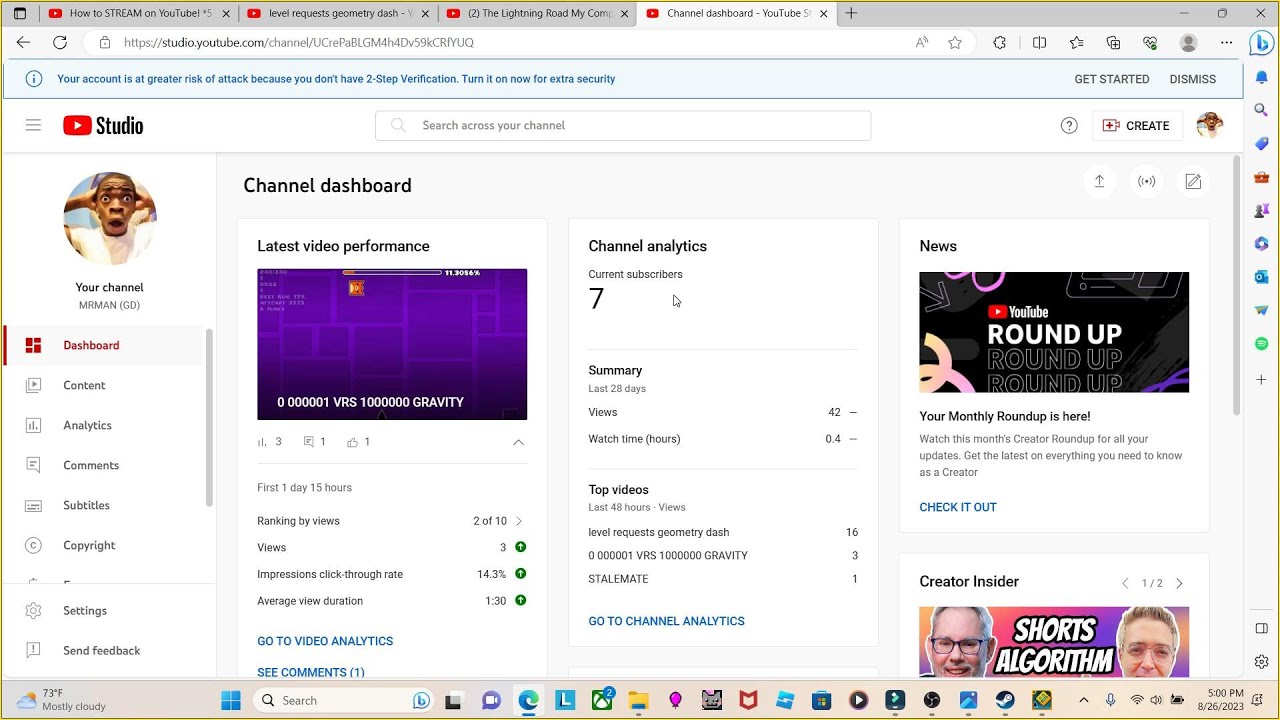The webpage displayed on a computer screen primarily consists of a user account alert and various navigation options for managing a YouTube channel. At the top, several red-highlighted squares indicate different sections of the page. Prominently in blue text, an alert warns, "Your account is at a greater risk of attack because you don't have two-step verification. Turn it on now for extra security." To the right of this message are options to "Get Started" or "Dismiss."

Directly below, a red square with an arrow pointing right is labeled "Studio." Adjacent to this is an image of a young man with brown skin and short brown hair, his mouth slightly open, and eyes wide with excitement or anticipation. Below the image, the text reads, "Your Channel for the YouTube channel."

Underneath this, the interface displays various navigation options in red text: "Dashboard," "Content," "Analytics," "Comments," "Subtitles," "Copyright," "Settings," and "Send Feedback." In the bottom corner, the weather is noted as 75 degrees and mostly cloudy.

On the right side of the page, sections labeled "Last Video Performance" and "Channel Analytics" are visible, with a purple square highlighting the latter. The current subscriber count is listed as seven. Further down, under "News," a section titled "YouTube Roundup" enthusiastically declares, "Your monthly roundup is here!"